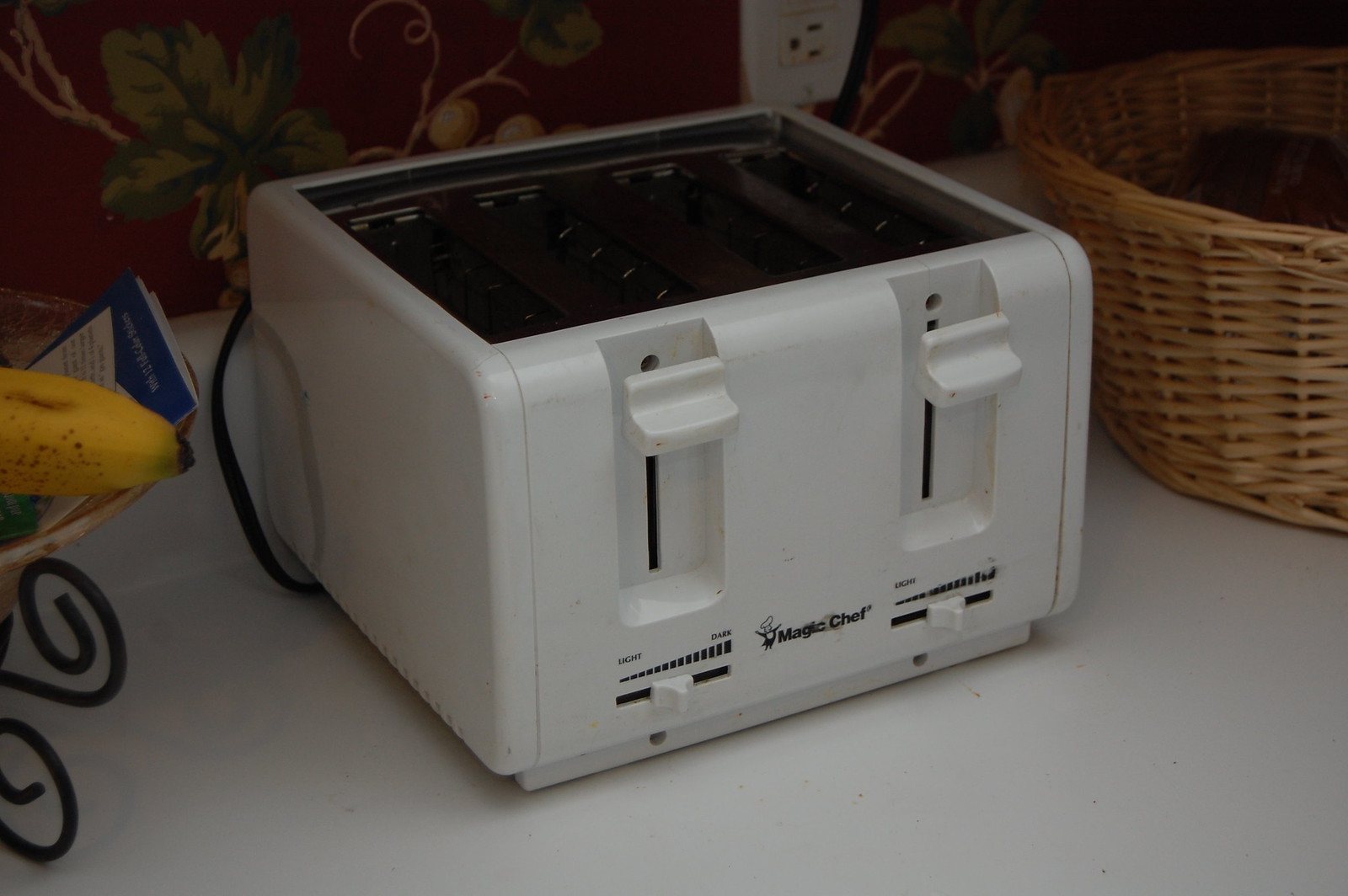In this color photograph taken in a kitchen, a central feature is the well-used Magic Chef toaster, which appears aged with some markings yet still functional. The toaster, white in color and capable of toasting up to four slices of bread, prominently displays the Magic Chef logo. It includes two knobs to lower the bread and two sliding buttons to adjust the toasting darkness for each pair of slots.

The toaster is positioned on a white countertop, and to the right, there's a wicker basket. To the left, a wrought iron basket contains a banana with dark brown spots and a hint of green at the tip. This basket also holds a few pamphlets. A white appliance plug is visible at the back of the counter, and the kitchen wall behind is adorned with maroon wallpaper featuring green leaves and beige fruit motifs.

This detailed setting highlights the practical and homey atmosphere of a busy kitchen.